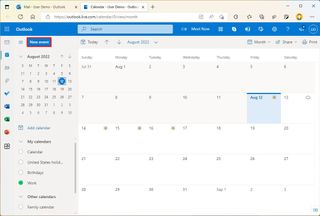This is a screenshot of a Microsoft Outlook calendar interface displayed within a browser window. The image is slightly blurry, rendering the text and numbers unreadable. The browser window, gray in color, shows two open tabs, one of which contains the Outlook calendar. 

At the top of the browser window, there is a blue search bar and a blue title bar featuring the barely visible word "Outlook" in white text. Below this, on the left-hand side, a minimized version of the calendar is displayed, while the main calendar occupies the right-hand side. The primary calendar view is predominantly black text on a white background, with one specific day highlighted in blue to indicate the current date of the screenshot. The screenshot appears to have been taken in August.

Along the left-hand sidebar, various colorful icons from the Microsoft Office suite are visible, including those for Word, Excel, and PowerPoint. The left-hand area also contains a grayed-out section, contributing to the overall structure of the Outlook interface.